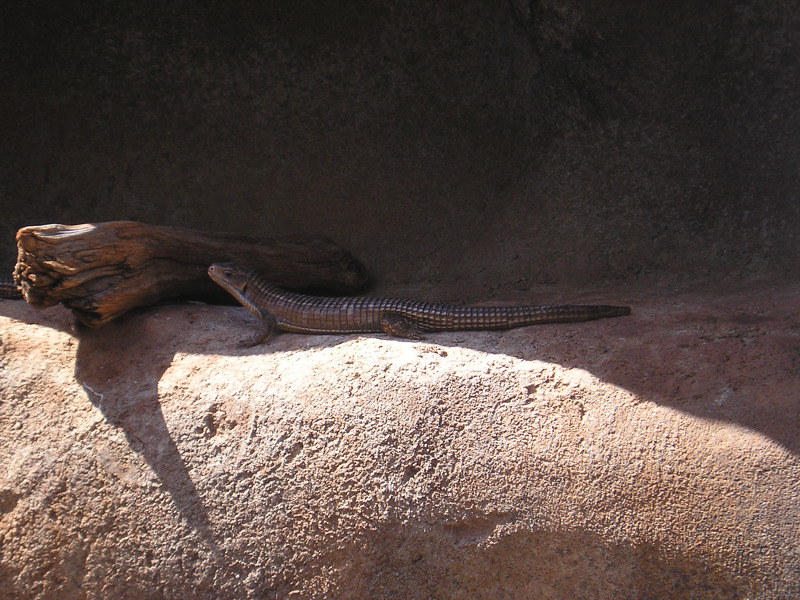The photo displays a small, brown lizard with a long, spiny tail and subtle whitish scales along its belly, lying leisurely on a rocky outcrop. Its front legs prop its upright head, while its back legs rest behind its body, giving an air of relaxation. In front of the lizard lies a rounded tree trunk, which appears large in comparison to the lizard. Just beyond the trunk, a glimpse of another similar tail suggests a second lizard of the same species. The scene appears to be within a rounded cave-like enclosure, with sunlight illuminating the lower portion of the outcrop while the lizard remains comfortably within the shaded area. The backdrop of dark brown rock contrasts with the sunlit, lighter rock in the foreground, enhancing the sense of depth in the enclosure, which could be part of a zoo exhibit or a natural desert habitat.